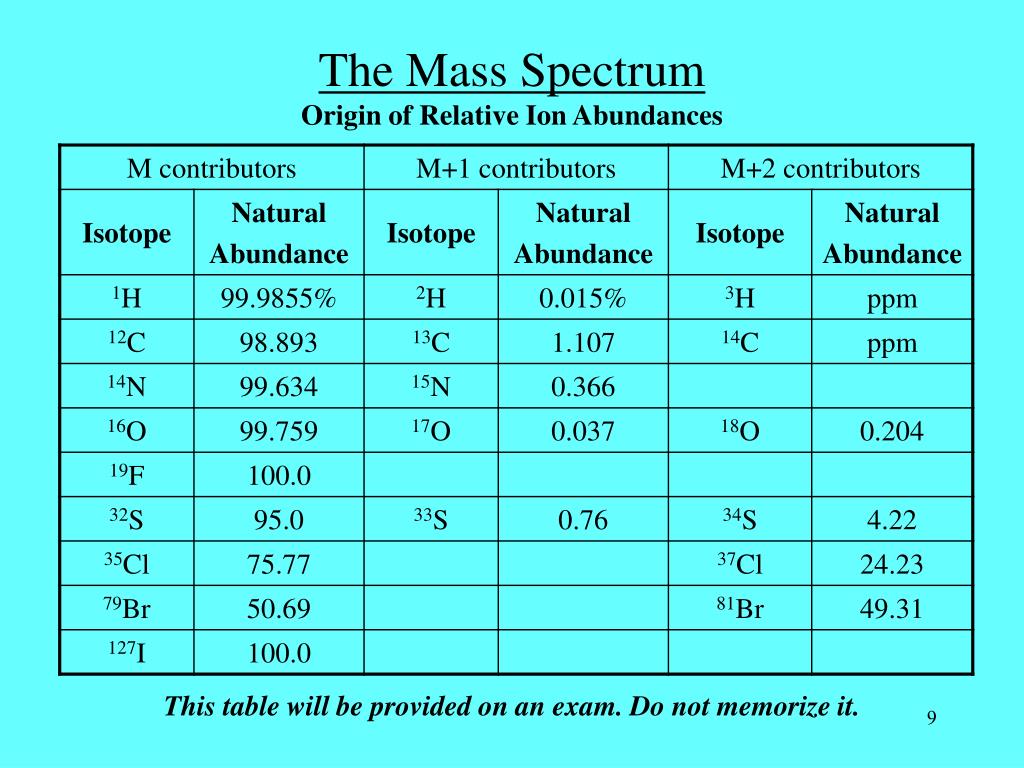The image displays a detailed table of data set against a light blue background, organized as a horizontal rectangle. At the top, the title "The Mass Spectrum" is underlined, followed by "Origin of Relative Ion Abundances," all in black Times New Roman font. The table is divided into three main columns titled "M Contributors," "M+1 Contributors," and "M+2 Contributors." Each of these columns is further divided into two sub-columns labeled "Isotope" and "Natural Abundance."

The elements listed under the "Isotope" sub-columns include:
- "M Contributors": 1H, 12C, 14N, 16O, 19F, 32S, 35Cl, 79Br, and 127I with corresponding natural abundances of 99.9885%, 98.893%, 99.634%, 99.759%, 100.0%, 95.0%, 75.77%, 50.69%, and 100.0%.
- "M+1 Contributors": 2H, 13C, 15N, 17O, and 33S with natural abundances of 0.015%, 1.107%, 0.366%, 0.037%, and 0.76%.
- "M+2 Contributors": 3H, 14C, 18O, 34S, 37Cl, and 81Br, where the percentages are given as PPM (parts per million) for some entries and specific values such as 0.204%, 4.22%, 24.23%, and 49.31%.

At the bottom of the table, a notice in italicized black text reads: "This table will be provided on an exam. Do not memorize it." Finally, the page number "9" is marked in the bottom right corner.